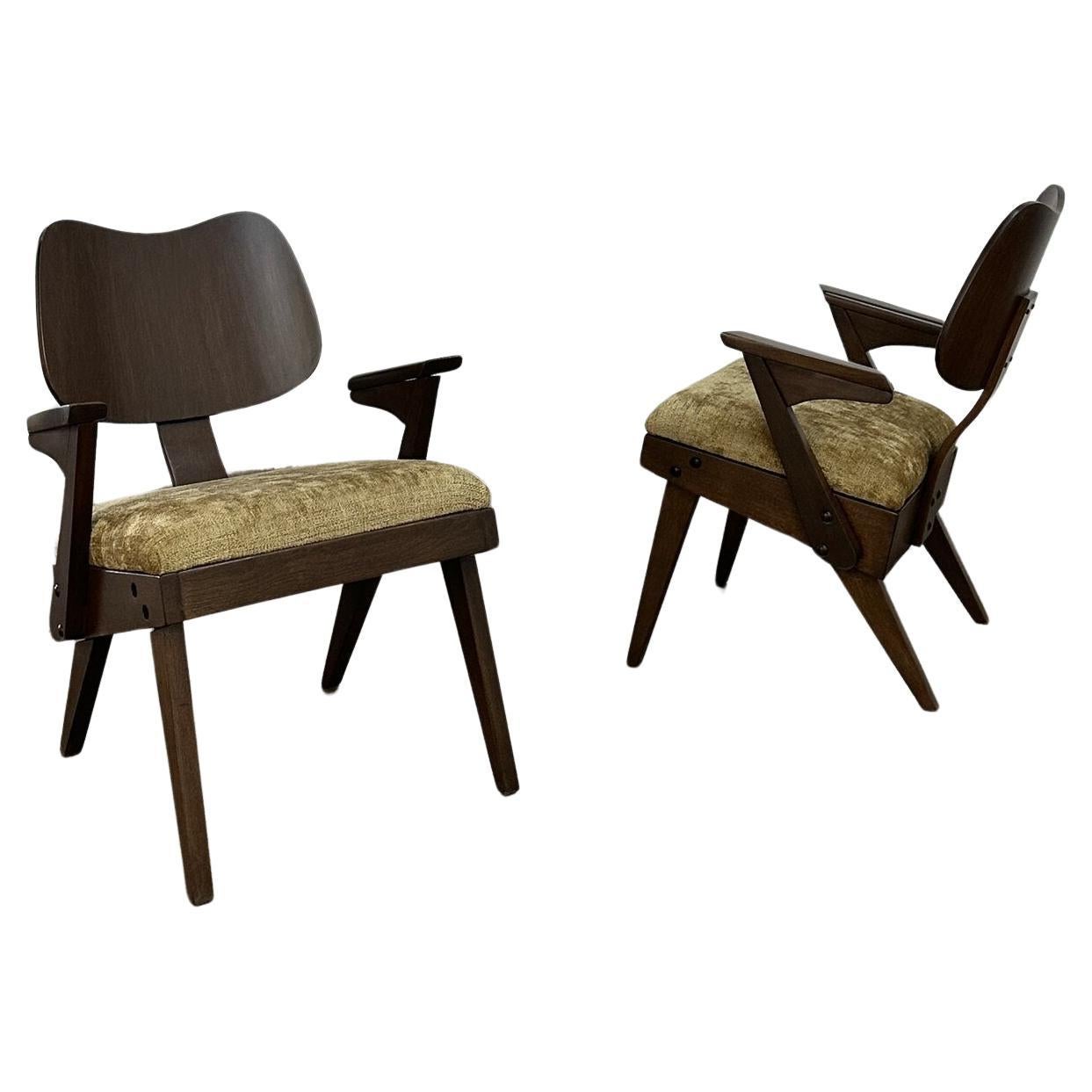This image features a pair of dark wood chairs that appear to be professionally rendered, possibly for a catalog or a furniture store's website, allowing customers to visualize them in their own spaces. Both chairs are characterized by low backrests and armrests, giving them an armchair-like quality, but they are versatile enough to function as dining chairs. Each chair is supported by four sturdy legs.

The chair on the left is displayed at a slight angle, offering a frontal view, while the chair on the right is shown from the side, providing a comprehensive look at its structure. Both chairs have a distinctive vintage feel, accented by straw-colored cushions that evoke a 1970s aesthetic. The cushions have a textured appearance, reminiscent of old-fashioned shag materials, adding a touch of retro charm to the overall design. These identical chairs, presented from different perspectives, showcase their elegant construction and nostalgic cushion design.